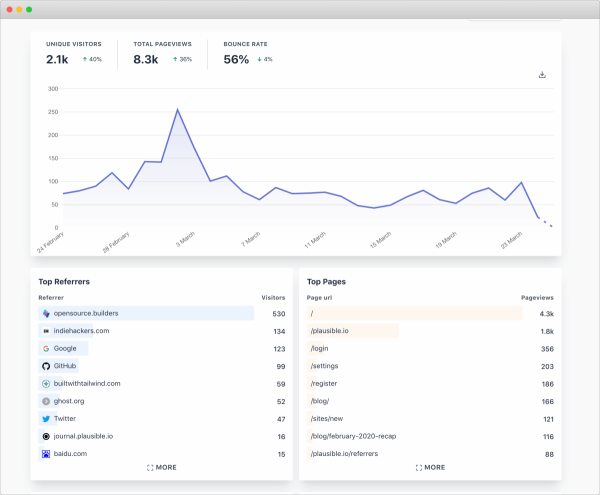**Screenshot Analysis of Website Dashboard Metrics:**

In the upper section of the screenshot, there is a light grey background typical of Apple’s interface, identifiable by the three traffic light circles in the top left corner—red, yellow, and green.

The dashboard is divided into two black rectangles containing key metrics. 

In the first rectangle:
- The text "Unique Visitors: 2.1k" is displayed in black with a green upward arrow indicating a 40% increase.

In the second rectangle:
- A vertical line separates the sections with "Total Page Views: 8.3k". This section has a green upward line but the specific percentage either reads "36%" or "30%". 
- Additionally, there's "Bounce Rate: 56%" with a green downward arrow indicating a 4% decrease.

The chart below this shows traffic trends with a vertical axis labeled with increments of 50 up to 300, and the dates range from February 24th to March 28th. A purple line indicates the data fluctuations over this period.

Below the chart, the "Top Referrers" section lists various sources such as Open Source Builders, Indie Hackers, Google, GitHub, and others. The corresponding visitor counts are 530, 134, 123, 99, 59, 52, 47, 16, and 15, respectively.

At the bottom of the screen, another section titled "Top Pages" presents a list of page URLs like `/login`, `/settings`, `/register`, `/blog`, `/site`, etc., with their respective page views: 4.3k, 1.8k, 356, 200, 186, 156, 121, 116, 88, and 77. The section ends with the option for "More".